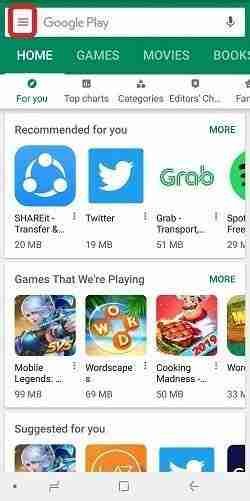This image captures the main screen of the Google Play Store, showcasing its interface in detail. The focus is on the hamburger menu icon in the upper left corner, which is highlighted in an unusual shade of green. This might be a customization by the user or a thematic change, possibly for St. Patrick's Day. The primary navigation bar at the top includes six tabs: Home, Games, Movies, Books, all presented in a familiar format.

Beneath these tabs, there are additional sections aimed at enhancing user experience, such as "For You," "Top Charts," "Categories," "Editor's Choice," all designed to help users discover new content. The "Recommended for You" section leverages AI to suggest apps based on user behavior and preferences.

Following this, a variety of games are displayed under the "Games We're Playing" section, indicating the user's varied interest in games. Finally, there's a "Suggested for You" category, although it's partially out of the visible screen area, hinting at more personalized recommendations just a scroll away.